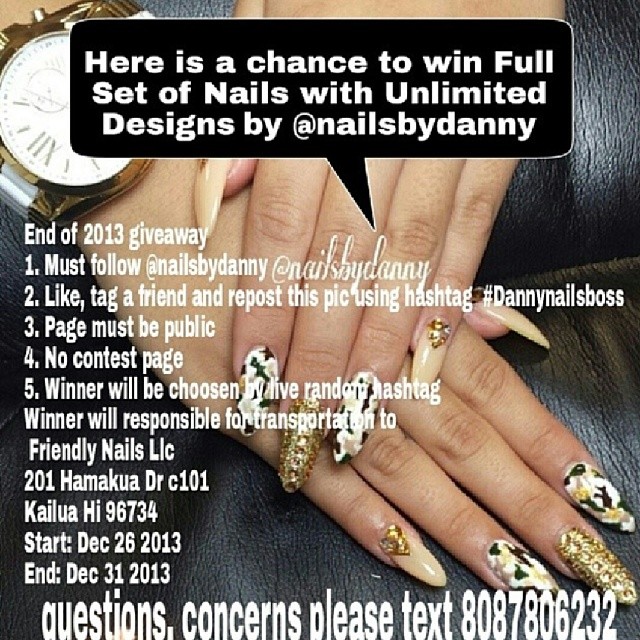This image is a detailed advertisement featuring a close-up photograph of a woman's hands with professionally done, elaborate fingernails. Each nail showcases a unique design with colors ranging from white to black, adorned with gold glitter and patterns. The woman is wearing a large gold watch on her right wrist, and her fingers are resting on what appears to be a leather purse. Overlaid on the photograph in white text, several instructions are provided for a giveaway promotion by Nails by Danny. The promotion offers a chance to win a full set of nails with unlimited designs. To participate, entrants must follow @NailsbyDanny, like, tag a friend, and repost the picture using the hashtag #DannyNailsBoss. The rules further specify that entrants' pages must be public, no contest pages are allowed, and the winner will be chosen via a live random hashtag selection. The winner is responsible for transportation to Friendly Nails LLC, located at 201 Hamakua Drive C101, Kailua, Hawaii, 96734. The giveaway runs from December 26, 2013, to December 31, 2013. For any questions or concerns, participants are encouraged to text 808-780-6232.